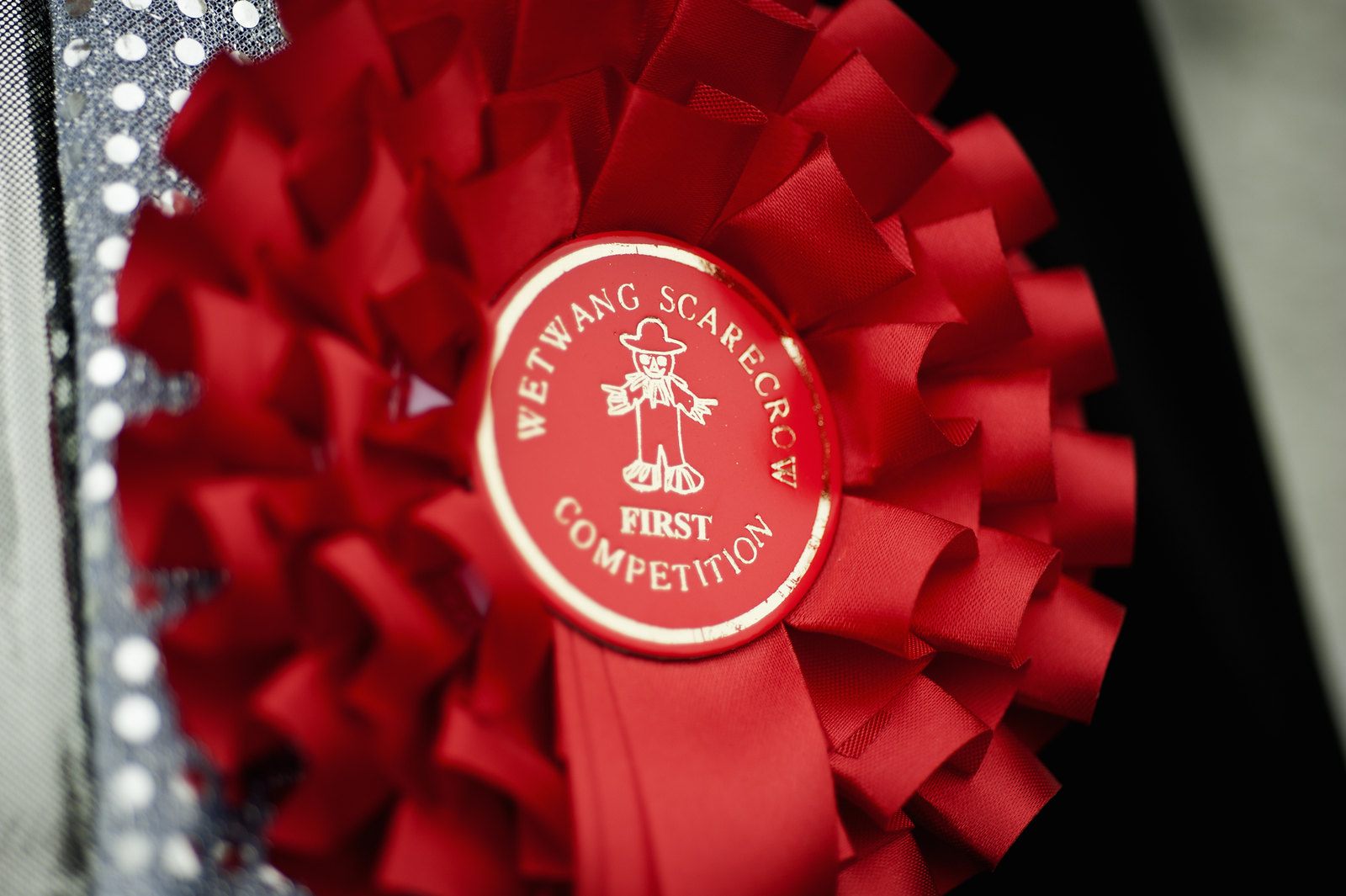This is a close-up photograph, approximately six inches wide and four inches tall, of a red and gold award ribbon, perfectly symmetrical and intricately designed. The award features a circular red center outlined in gold. At the core is a golden scarecrow, adorned with a hat and possibly red pants. Surrounding the scarecrow, in gold capital letters, the text reads "Wet Wang Scarecrow" on the top arc and "First Competition" on the bottom arc, arranged such that the letters form slight arches. 

Encircling the central medallion, the ribbon forms several layers of curved, red loops that create a flower-like effect. These loops increase in size from the center outward, adding volume and texture to the ribbon. Below the main circular part of the ribbon, a single red tail hangs down, matching the ribbon's central theme.

The background of the image is a contrast between two distinct sides. On the left, there's a silvery, glittery fabric with rows and columns of small silver dots, possibly part of a handbag. On the right, a black, diagonally slanted background meets a blurred gray area, providing an elegant backdrop to the vivid award ribbon. The entire scene conveys a sense of pride and achievement, typical of a prized ribbon one might win at a prestigious competition.